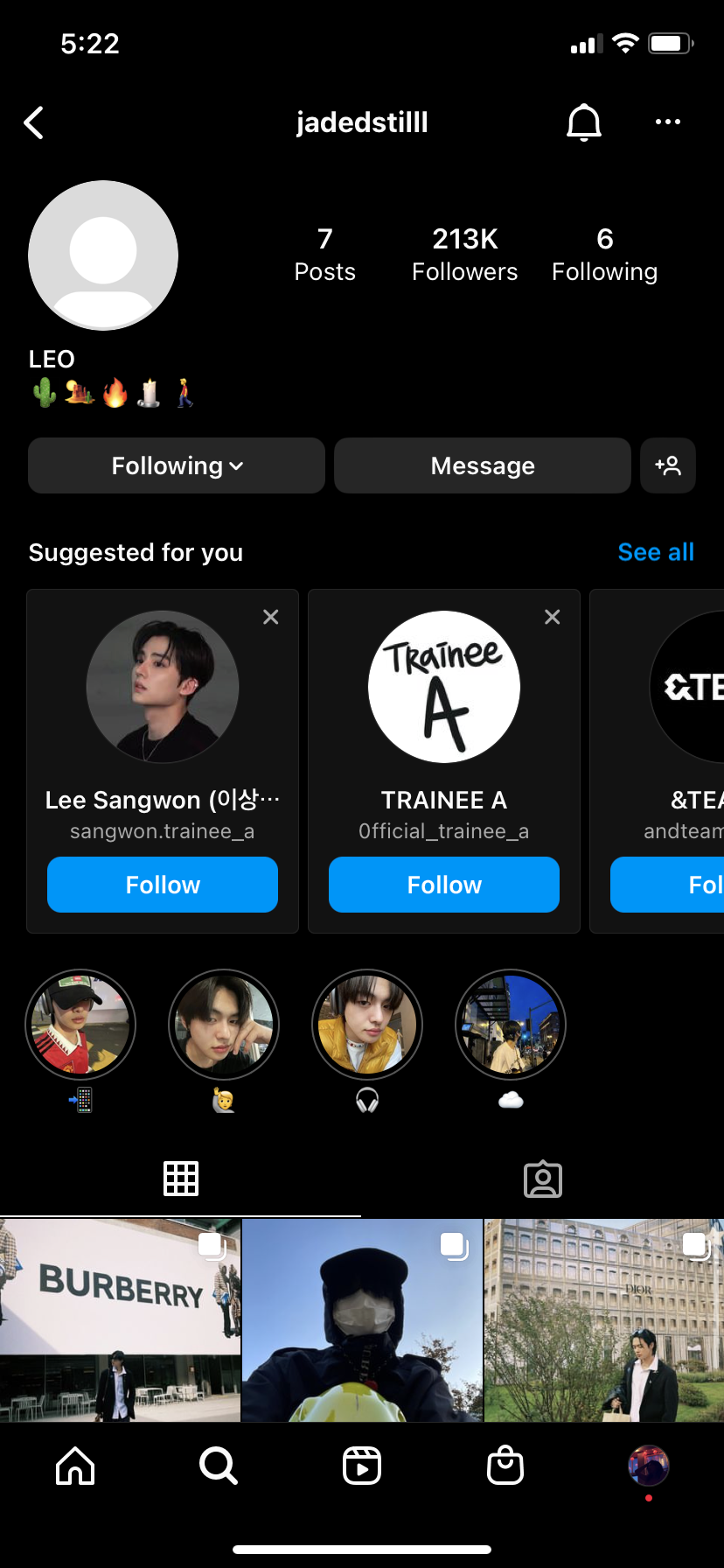The image features a social media profile header displaying several icons, including a Wi-Fi signal, battery indicator, and a back arrow. The user has the handle "jaded still" and the profile status notes a grey circle. The profile summary shows 7 posts, 213k followers, and 6 following, with the bio containing the words "Leo" and "Cactus." There is an option to follow or send a message, and a "Suggested for you" section listing "Lee Sing Wong" and "trainee A, official trainee A," both highlighted in blue.

Beneath this profile information, the main image displays a person in a red shirt with short hair wearing a yellow vest, standing against a backdrop of a blue sky with scattered clouds. The image composition includes a grid-like pattern with squares overlaying the scene, featuring various elements such as the person's head adorned with a Burberry accessory, glimpses of distant buildings and houses, and other icons like a magnifying glass, play button, and shopping cart, some of which are highlighted in purple.